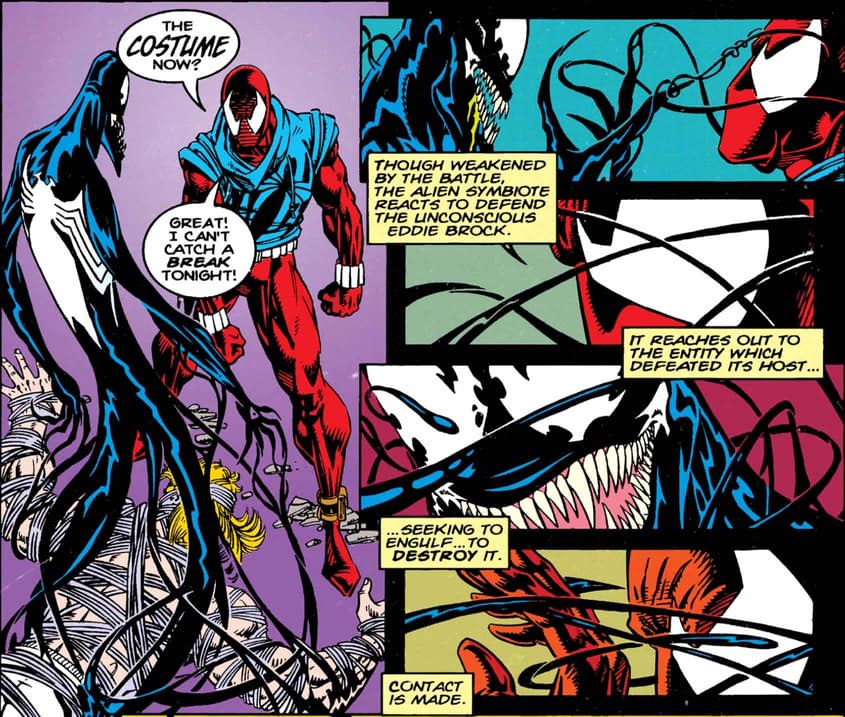The image depicts a vibrant and intense comic book scene featuring a confrontation between a man in a blue top, with red arms, legs, and mask, and a blue and black creature with a very long tail and long nails. On the left side of the page, the man in the red mask faces the creature, who appears to be Venom, standing over someone tied up and unconscious. The dialogue bubbles show the man in red saying, “The costume now? Great, I can't catch a break tonight.” 

The right side of the page is divided into four smaller panels: 

1. **Top Panel**: A close-up of both the man and the creature’s faces, showcasing their intense expressions.
2. **Second Panel**: Focuses solely on the superhero.
3. **Third Panel**: Features the villain alone, presented in a striking pose.
4. **Bottom Panel**: Illustrates an action moment, possibly the creature striking or making contact with the superhero. The narrative box narrates, “Though weakened by the battle, the alien symbiote reacts to defend the unconscious Eddie Brock. It reaches out to the entity which defeated its host. Seeking to engulf, to destroy it, contact is made.”

The backgrounds of these panels are distinctly colorful, transitioning through blue, green, red, and yellow from top to bottom, enhancing the dynamic and dramatic nature of the artwork. The overall style is unmistakably comic book-like, with bold colors, action-packed compositions, and dramatic text.